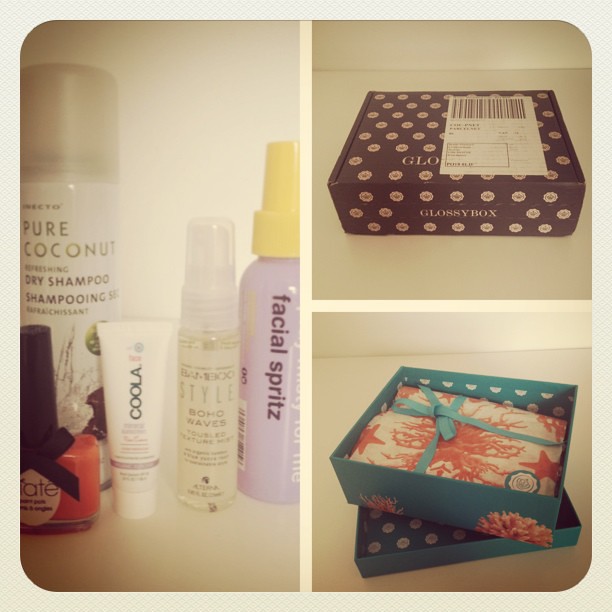The image features a wellness or beauty gift box displayed in a catalog-style layout with a gray background. It is composed of three photographs, arranged in a square with rounded corners: a vertical rectangle on the left and two squares stacked on the right. 

On the left side, various beauty and skincare items are neatly arranged on a gray countertop. Prominently displayed is a large white spray container labeled "Pure Coconut Dry Shampoo," though some text is blurry and unreadable. Below it is a pink liquid product, possibly nail polish, with a long black lid. Adjacent to this is a white squeeze tube labeled "Koola," though the rest of the text is out of focus. Further right, there's a clear spray bottle with the word "Bonsaver," and another purple facial spritz spray bottle with a yellow lid.

To the right, the upper image showcases a black gift box adorned with white and light purple polka dots. The bottom image features a light blue gift box with a floral print, shown lying open to reveal a flat red and white package tied with a blue ribbon. 

Overall, the detailed product display, organized presentation, and specific descriptions suggest a catalog designed to highlight the appealing aesthetics and variety of the gift items.